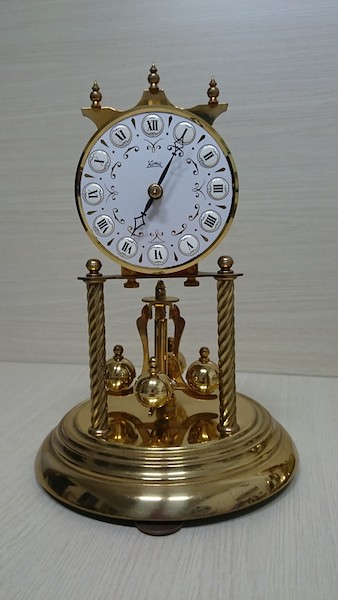This photograph features a small gold tabletop clock in stunning crystal-clear quality. The clock rests elegantly on a white wood surface, which matches the white wood wall serving as the backdrop. The clock's design is finely detailed, beginning with its rounded gold base, which supports two slender gold columns on either side. Nestled between these columns are three small gold orbs, adding a touch of sophistication.

The clock's body is encircled with a gold frame, encapsulating a pristine white clock face adorned with what appears to be dark brown, possibly black, Roman numerals. The hour and minute hands are similarly dark brown, providing a striking contrast to the white background. A gold circle marks the center of the clock face, drawing attention to its precise craftsmanship.

Crowning the clock are intricate spiky gold designs, adding a regal flourish to the timepiece. Soft light reflects off the bottom of the clock, accentuating its polished finish and enhancing the overall elegance of the scene.